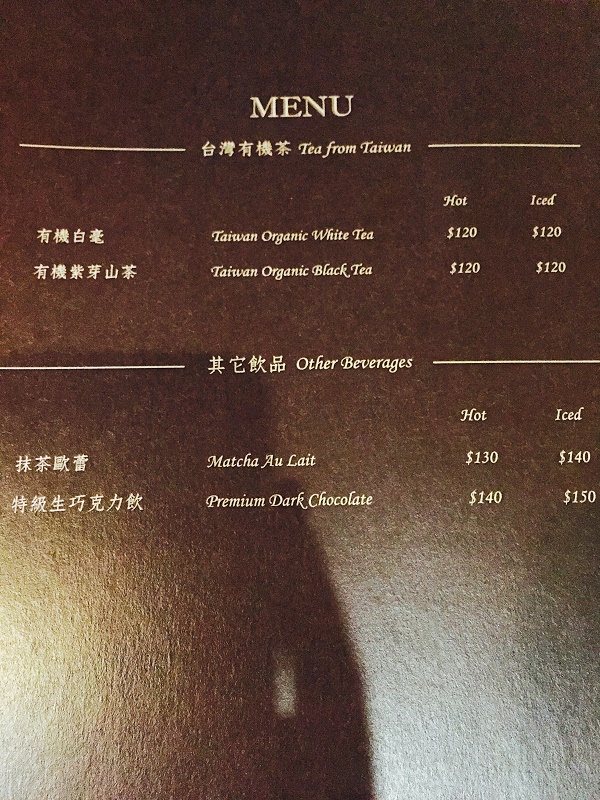The image captures a detailed menu from a Chinese or Taiwanese tea shop, presented on a brown background. The menu is divided into two main subheadings: "Tea from Taiwan" and "Other Beverages," each accompanied by both English and Chinese characters. Under "Tea from Taiwan," two items are featured: Taiwan Organic White Tea and Taiwan Organic Black Tea. The "Other Beverages" section lists Matcha Ole and Premium Dark Chocolate. Pricing for each item is indicated for both hot and iced options, displayed on the right side, and notably lacks decimal points, suggesting this menu might be from abroad. The menu layout positions Chinese characters on the far left, English translations in the center, and pricing on the right.